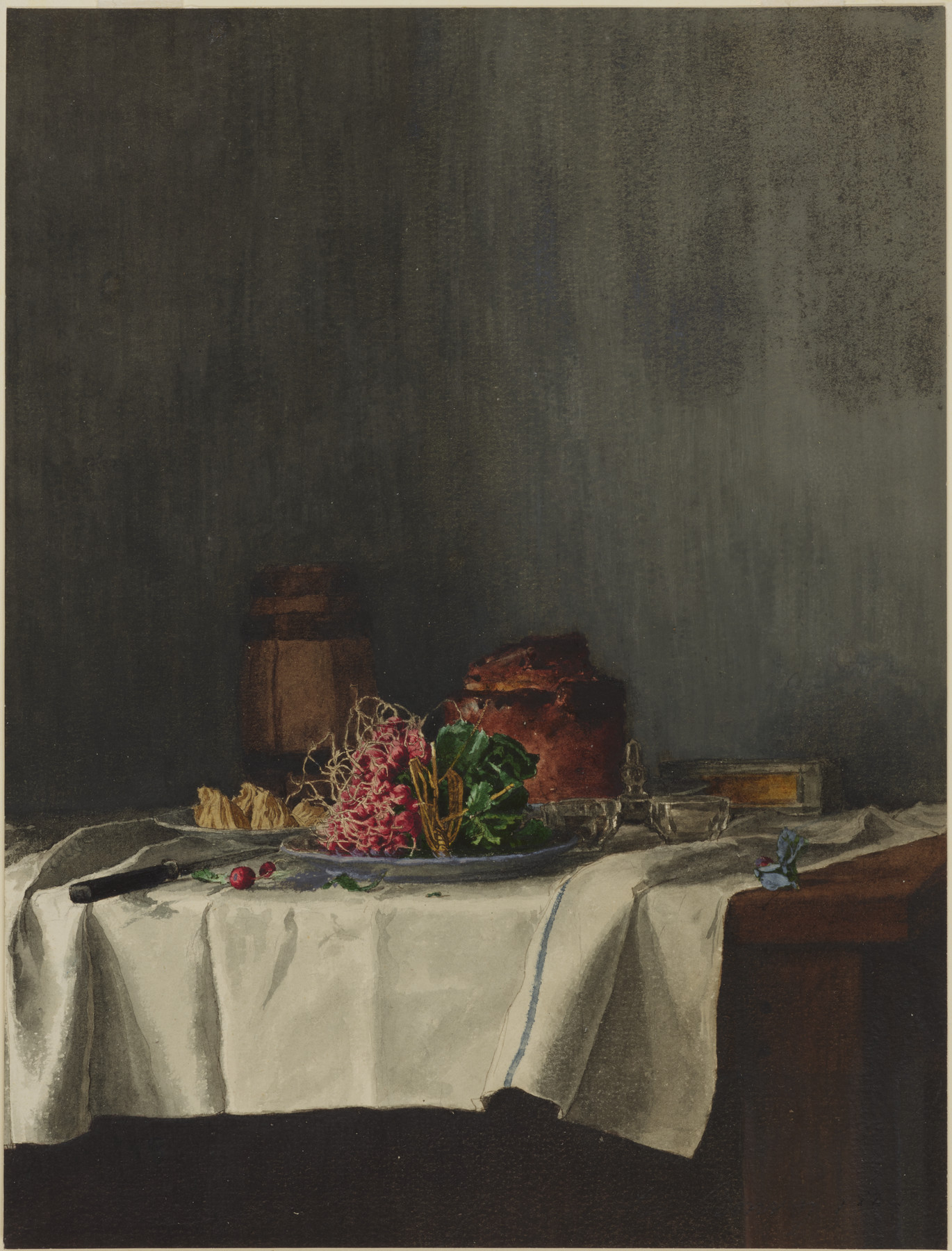This artistic painting, rendered within a vertically-aligned rectangular frame, features a rustic scene that seamlessly blends shades of brown and grey. The background, a wall with vertical lines of alternating light and dark browns and fading grey shades, provides a subtle contrast to the foreground elements. Dominating the lower half of the painting is a rich mahogany wooden table, dynamically aligned with a slight diagonal tilt, higher on the right. Draped casually over a portion of the table is a rectangular, white tablecloth, gently folded on the right side and characterized by a blue stripe.

Prominently placed on the table are several notable objects: a large silver platter on the right, brimming with green leaves, pink radishes, and possibly some yellow dry flowers, indicating a salad arrangement. Adjacent to these, rough tan cookies or possibly bread provide a rustic touch. Adding to the setting are two cylindrical, reddish-brown wooden barrels or pots situated at the table's back, and a clear plate hosting a round loaf of freshly baked bread, slightly burnt at the edges for an authentic feel. 

Enhancing the scene's detail, small round, empty glass dishes are scattered across the table, with a blue floral element adding a delicate touch near the edge. A kitchen towel or tablecloth, partway draped over the front of the table, reveals its white expanses and dark brown underside, while a knife lies casually on the table. The dark brown color of the table’s front base further grounds the entire composition, adding depth and dimension to this finely rendered, potentially antique scene reminiscent of professional artwork.